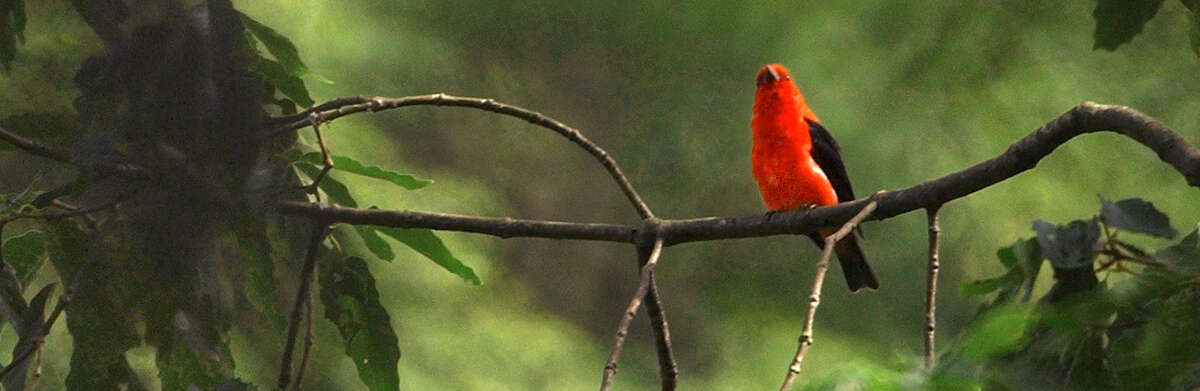In this panoramic, sunlit outdoor photograph, a striking bird, likely a cardinal, commands attention as it sits on a thin, elongated branch that stretches horizontally across the image from left to right. The cardinal’s vibrant red plumage contrasts with its black wings and tail feathers, and its golden beak is prominent as it faces towards the camera. The background, while blurred, is a lush tapestry of various shades of green, suggesting a verdant, wooded setting. The branch the bird perches on is adorned with several elongated leaves, with denser foliage appearing towards the left side of the image and sparse leaves on the right. The natural light highlights the bird’s vivid belly and throat, adding a dynamic contrast against the leafy backdrop.